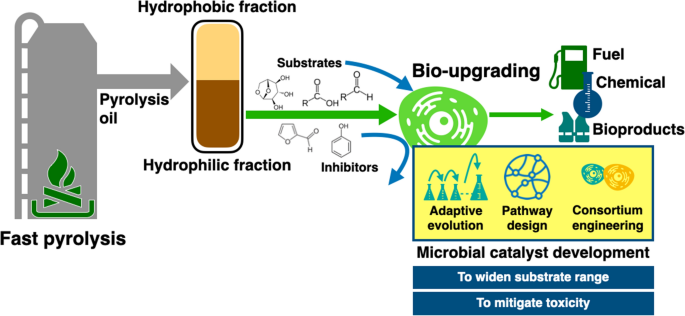The infographic depicts a detailed diagram of a scientific and chemical process associated with fast pyrolysis in a gray silo. On the left, the gray silo features a green flame symbolizing pyrolysis oil, with a ladder on the left side of the tank. A gray arrow from the silo points to a capsule-like image, tan on top and brown on the bottom, labeled "hydrophobic fraction," and beneath this, another label reads "hydrophilic fraction."

Adjacent to this, a green arrow directs attention to a green circle divided into sections marked "substrates" (at the top, with three different chemicals) and "inhibitors" (below). Above the green circle, the term "bio-upgrading" is noted, with a blue arrow indicating a catalytic process. Further to the right, another green arrow leads to an image of a gas pump and other icons signifying "fuel," "chemical," and "bioproducts."

Below this main section, a smaller infographic details intermediary steps, featuring a yellow box labeled "adaptive evolution," a blue circle marked "pathway design," and two smaller circles indicating "consortium engineering." Outside of these, blue text states "microbial catalyst development." Additionally, two long rectangles, separated by white lines, contain white text stating goals: the first rectangle aims "to widen substrate range," while the second aims "to mitigate toxicity."

All these elements are set against a plain white background, keeping the focus entirely on the diagrammatic content.